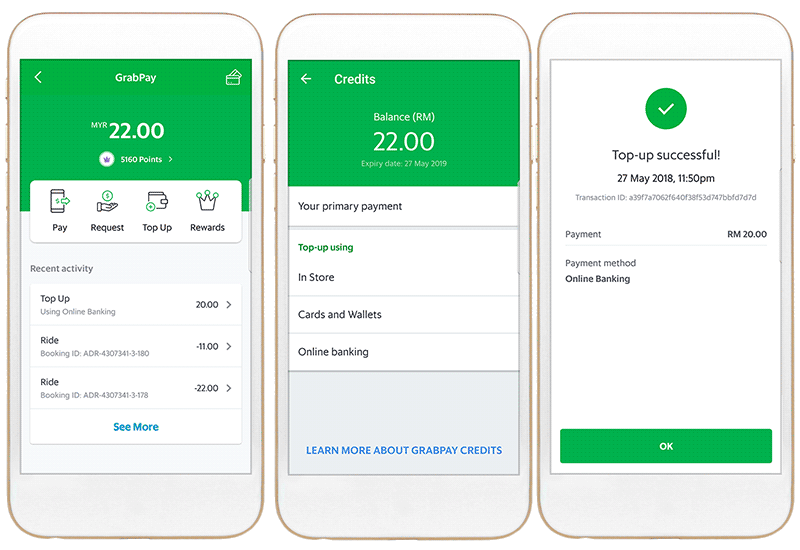The image is a composite of three individual smartphone screenshots with a gray outline indicative of the phone case. Arranged from left to right, the screenshots showcase various screens of the GrabPay app.

**First Screen (Leftmost):**
- **Header:**
  - A broad emerald green section at the top.
  - "GrabPay" is displayed in white text.
  - Below it, "MYR $22" (Malaysian Ringgit) also in white, followed by "5,160 points".
  - A small purple crown icon with a white circle to its left.

- **Main Content:**
  - Icons and Text:
    - An icon resembling a cell phone above the word "Pay".
    - A handout icon with a dollar sign above "Request".
    - A wallet icon with a green plus sign symbolizing add funds.
    - A black crown with green dots on the points, labeled "Rewards".

- **Recent Activity Section:**
  - "Recent Activity" in bold text.
  - Transactions listed:
    - "Top Up $20",
    - "Ride $11",
    - "Ride $22".
  - A blue "See More" text at the bottom.

**Second Screen (Middle):**
- **Header:**
  - Similar emerald green section.
  - Displays "RM Balance" (Ringgit Malaysia).
  - "Credits" in white text at the top left.
  - Below it, "Expiry Date 27 May 2019".

- **Main Content:**
  - Black Text:
    - "Your Primary Payment".
    - "Top Up Using" in green text.
  - Options in black:
    - "In-Store",
    - "Cards and Wallets",
    - "Online Banking".

- **Footer:**
  - A bold, cornflower blue line displaying "Learn More about GrabPay Credits".

**Third Screen (Rightmost):**
- **Header:**
  - A green circle with a white checkmark.

- **Main Content:**
  - Black text on a white background:
    - "Top Up Successful 27 May 2018, 11.50pm".
    - "Transaction ID", followed by an alphanumeric code.
  - Transaction Details:
    - "Payment: RM $20".
    - "Payment Method: Online Banking".

- **Footer:**
  - A long horizontal green bar with "OK" in white text.

The screenshots illustrate different functionalities of the GrabPay app, from balance and rewards display to successful transaction confirmation.